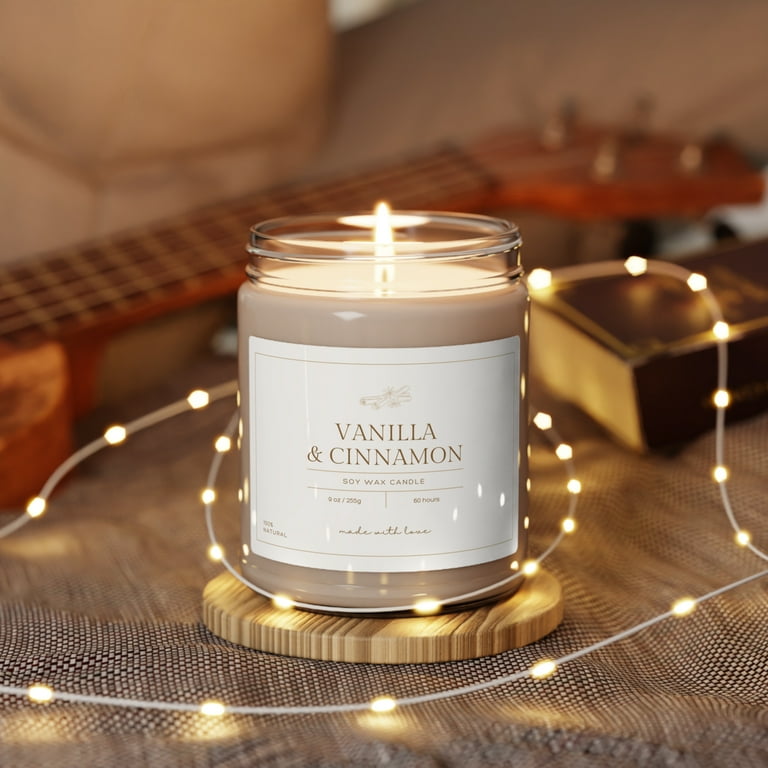A warm and cozy scene is captured in this image, featuring a lit soy wax candle housed in a glass jar. The candle, which emits a soft glow, has a serene light beige or dark tan wax and a small, flickering flame. On the front of the jar, a white label in brown font reads "Vanilla and Cinnamon," indicating the fragrance. The jar is placed atop a circular, light-brown wooden coaster. Delicately wrapped around the jar and spilling out of frame are small, glowing fairy lights. In the softly blurred background, a homely living room comes into view, showing the head of an acoustic guitar, a couch, and a book resting on a table. The ambiance is inviting and warm, suggesting this image could serve as an advertisement for the candle, highlighting its natural ingredients and loving craftsmanship. The photo also provides useful details such as the candle's weight of 9 ounces (255 grams) and a notable burning time of 60 hours.